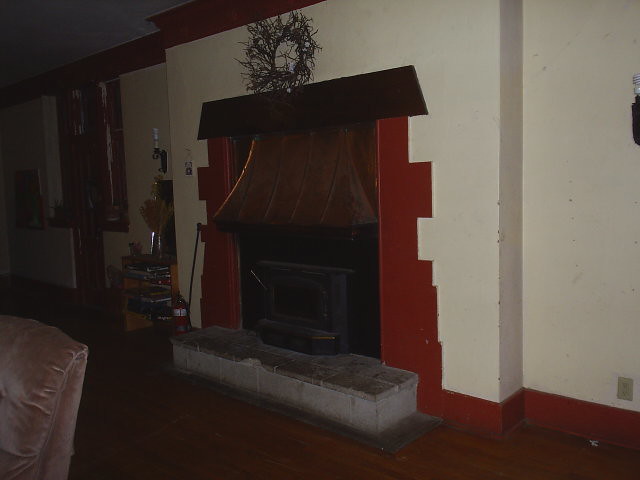The photograph, taken in dim lighting with a flash, depicts a living room in an old, weathered house. At the center is an aged, inactive fireplace with a chipped and almost black concrete hearth and an iron insert. Above the fireplace is a tin roof-like structure and a thin, dried wreath made of branches. The white walls surrounding the fireplace are heavily marked with black smudges, scrapes, and chips, indicating neglect. Red baseboards extend into the siding of the fireplace, framing it along with a brown-painted top section that mimics a small house facade. 

The room is cluttered, with partially visible items such as books or records, a small piece of a brown sofa, a chair, and some board games to the left of the fireplace. Additionally, there are hardwood floors and a window faintly visible in the background. The entire scene suggests a neglected, dirty interior that could benefit from significant maintenance.